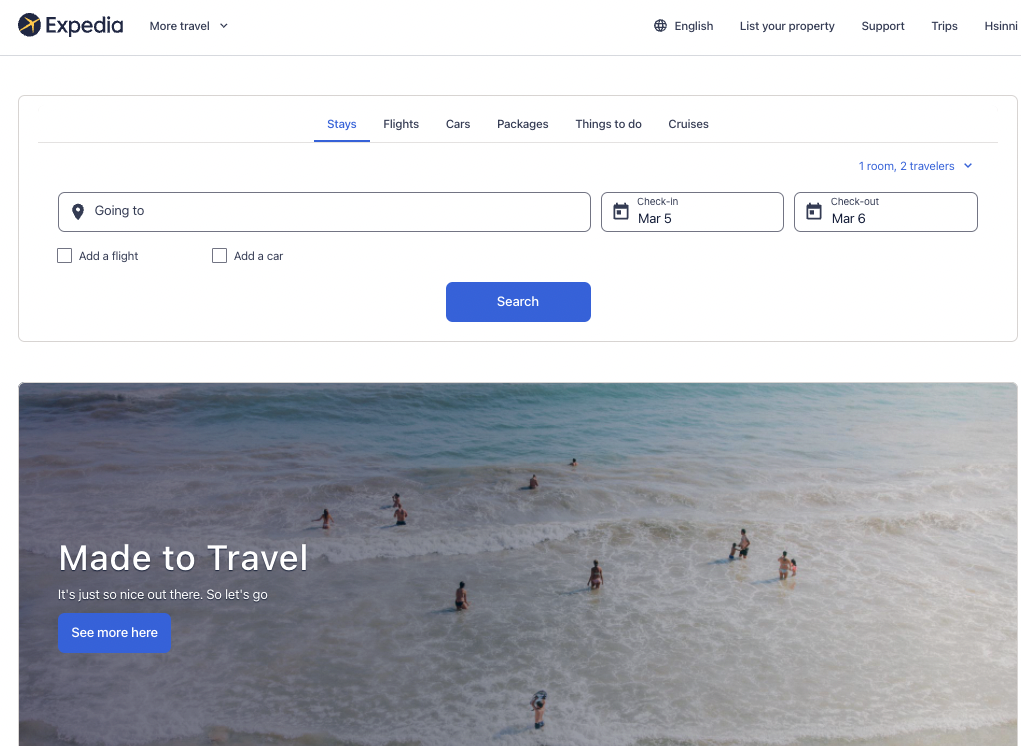The image captures a screenshot of the Expedia website, specifically the desktop version. The layout is simple and clean, dominated by a white background. At the top of the screen, the Expedia logo is prominently displayed, along with the text "More Travel" and a language selector set to English. The navigation bar includes options such as "List Your Property," "Support," "Trips," and an account name that appears to be "Hisini."

Below the navigation bar, there are several interactive options for users to plan their trips, including tabs for "Stays," "Flights," "Cars," "Packages," "Things to Do," and "Cruises." Central to the interface is a search bar with fields for destination entry ("Going To"), and options to add a flight or car. Users can also specify check-in dates, the number of rooms, and the number of travelers.

Further down, the website features a visually appealing photo of a beach, showcasing travelers joyfully frolicking in the ocean. Superimposed on the image is the motivational phrase "Made to Travel," encouraging potential travelers to explore more destinations. This section seems to invite users to learn more about enticing travel opportunities.